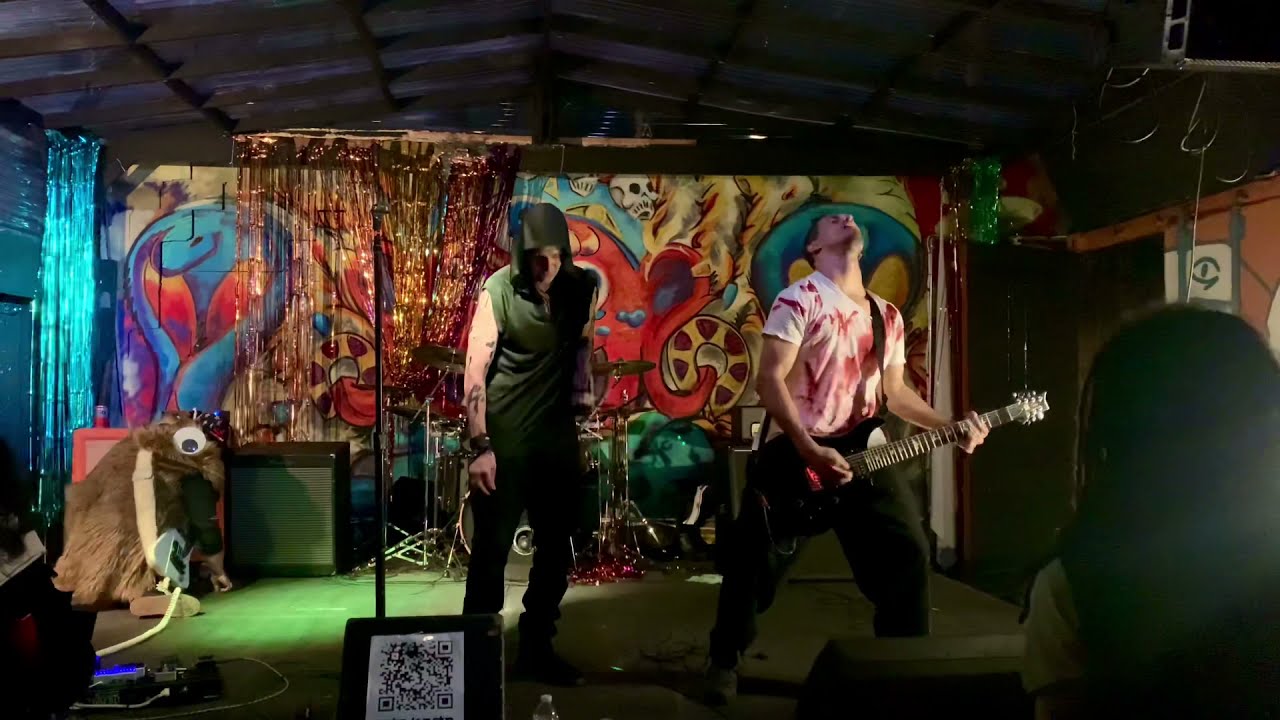This photograph captures a rock band performing on a small, dingy stage in what appears to be a garage or nightclub. The stage, notably green-floored, is littered with vivid elements: a backdrop adorned with graffiti-style murals featuring a blue cobra, a skull, a red octopus, a film reel, and various psychedelic shapes in swirling colors of red, blue, yellow, orange, pink, and purple. On the right, the lead guitarist, clad in a striking tie-dye shirt resembling blood splatters and black pants, thrashes his black electric guitar, head thrown back in the throes of music. Beside him stands the lead singer, dressed in a sleeveless green tank top hoodie, black pants, and displaying tattoos on his bare arms. His black hair tumbles over his face as he gazes downward. A drum kit sits behind them, obscured by the lead singer. The left side of the stage is cluttered with hanging beads, tall black speakers, and amplifiers, contributing to the dark, gloomy ambiance. At the very edge of the image, the faint outline of a woman in shadow is visible, identifiable only by her dark hair and gray shirt. A QR code sign with a black rim and furry, eye-topped props add quirky details that accentuate the makeshift, rundown venue aesthetic.